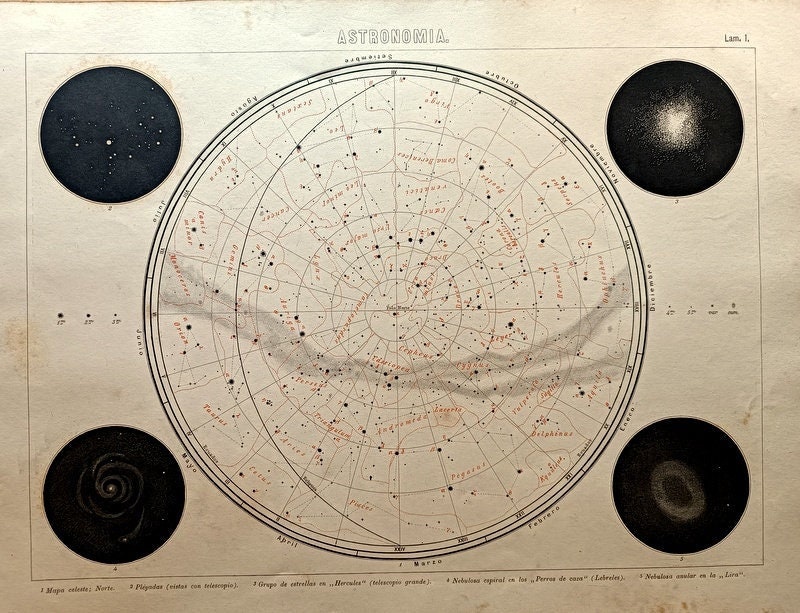The image is of a vintage celestial map titled "ASTRONOMIA" at the top, printed on aged, brownish paper with smudges of light pink and gray hues, giving it an antiquated appearance. At the center, there is a large circular diagram resembling a radar with intricate black outlines and red text, including numerous black dots and a web of lines forming grids and curvatures. Radiating from the center are lines that create various divisions of the celestial bodies, surrounded by annotations of degrees, months, and other labels that are faint and difficult to read due to their tiny, cursive font.

Around this central circle are four smaller black circular insets located at each corner of the image—upper left, upper right, lower left, and lower right. The upper left circle showcases scattered white dots resembling distant stars, while the upper right circle features clustered dots in the center. The lower left has swirled patterns of light, and the lower right contains an oval-shaped white light fading outwards. Additional unclear text appears at the bottom of the map, and the terms "lamb one" or similar can be found on the top right corner of the page. This detailed celestial map appears to illustrate astronomical phenomena and constellation structures, encapsulated in a meticulously drawn and labeled format.